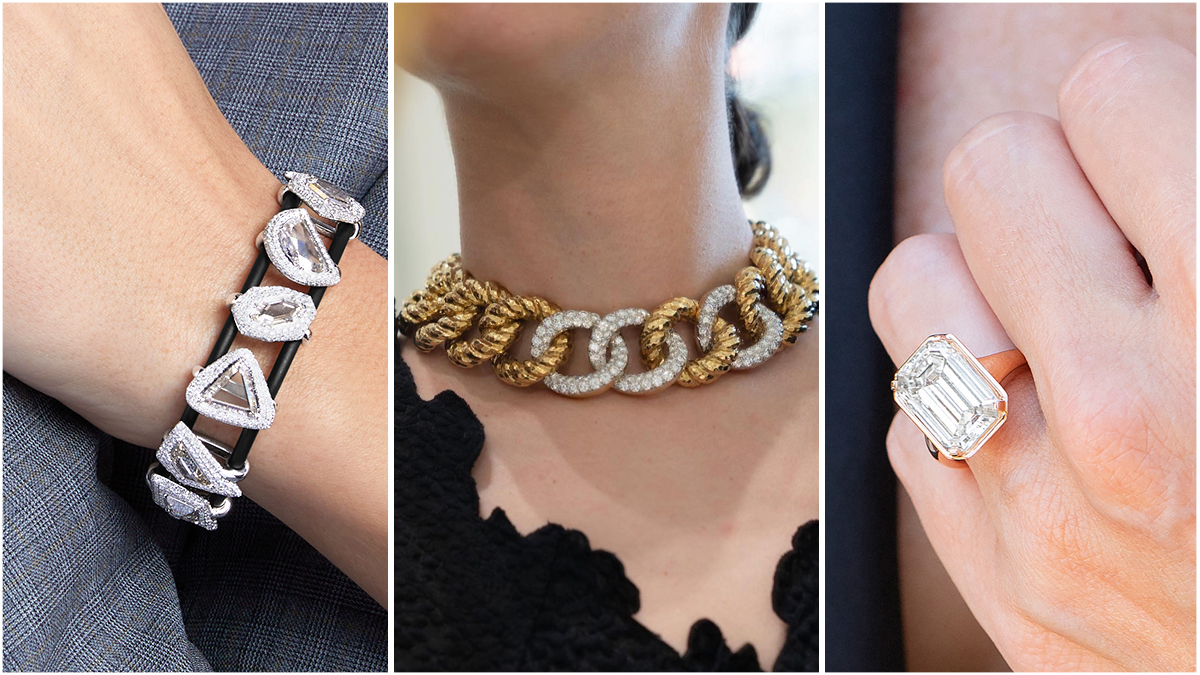This image compilation appears to be an advertisement for a jewelry brand, showcasing three detailed photographs of elegant jewelry pieces. In the left photograph, a woman is shown against a sweet suit, modeling a striking black and silver bracelet adorned with various shapes that could be diamonds or other precious stones. The central photograph captures a woman wearing a bold, chain-like necklace composed of alternating large gold and silver links. The woman is dressed in a black ruffled v-neck dress with her hair pulled back, highlighting the necklace's intricate design, which includes rings that could be set with large diamonds. The right photograph features a close-up of a woman’s hand adorned with an ornate gold ring, set with a large, clear, square-oval shaped stone that could be a diamond, though it resembles high-end costume jewelry. The overall color palette of the image includes flesh tones, gold, silver, and touches of black, contributing to a sophisticated and luxurious aesthetic.